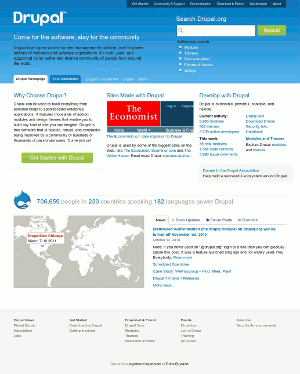A small screenshot of a Drupal website is shown. At the top, there's a dark blue-black navigation bar with text that's difficult to make out. Below this bar, a lighter blue section houses a prominent white search bar with a green button labeled "Search for Drupal.org." Under the search bar, faintly visible text is present. On the left-hand side of the page in larger white letters, the text reads: "Drupal: Come for the code, stay for the community." A world map is situated at the bottom left, featuring white continents on a gray ocean background. Above the map, blue text states "706,569 people," followed by gray text, then "230 countries speaking," in blue, "182 languages," in gray, "power Drupal." Some menus and selections at the bottom are blurred and illegible. Additionally, there appears to be an advertisement from The Economist, which features white lettering on a red background and is located at the upper middle section of the page.